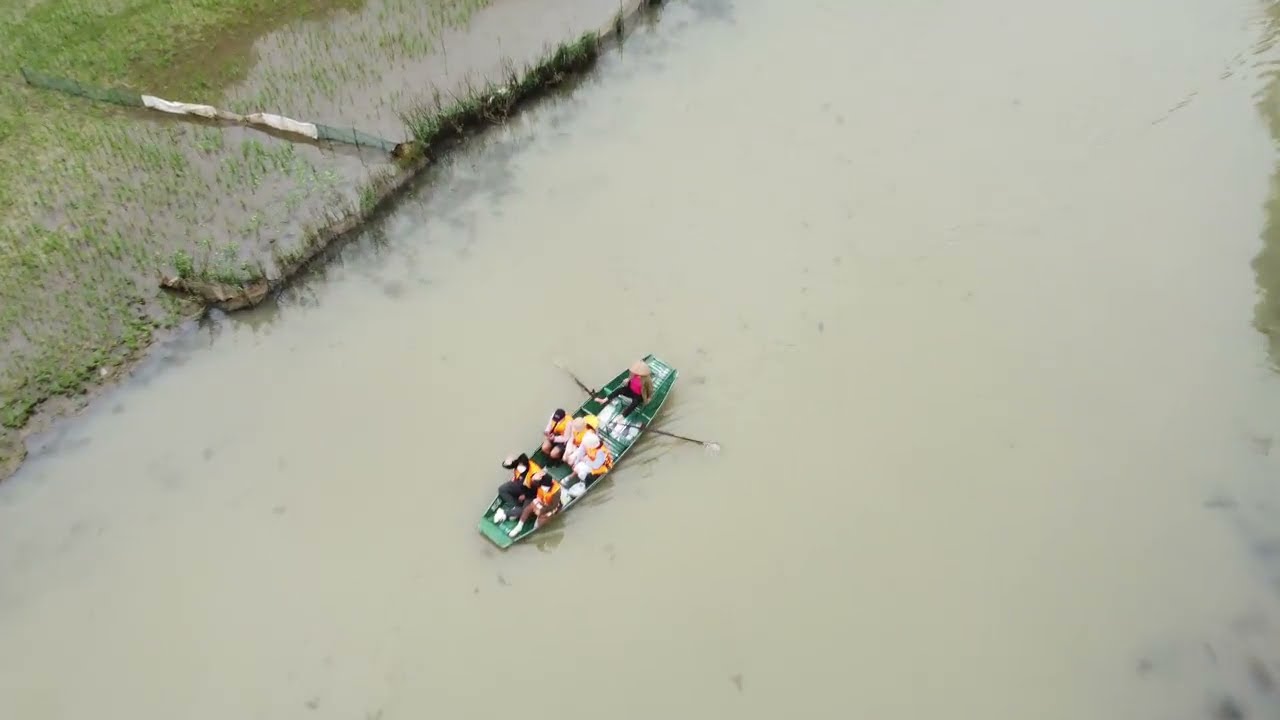This detailed aerial view captures a murky green and brown river alongside a flooded rice paddy located in the upper left corner of the image. The paddy is divided by a green and white fence, creating a distinct separation within the agricultural area. Predominantly green and brown, the river hosts a small, green rectangular paddle boat accommodating six passengers. Five of these tourists are dressed in casual clothing with baseball caps and orange life vests, visibly seated in two rows of three on orange benches. The individual steering the boat, positioned at the back next to two black and white paddles, is distinctly attired in a brown jacket, red shirt, black pants, and a traditional straw hat. Various white sacks can also be seen within the boat. Notably, the right side of the image reflects the silhouettes of several trees on the river's surface, adding a natural frame to this vibrant scene.